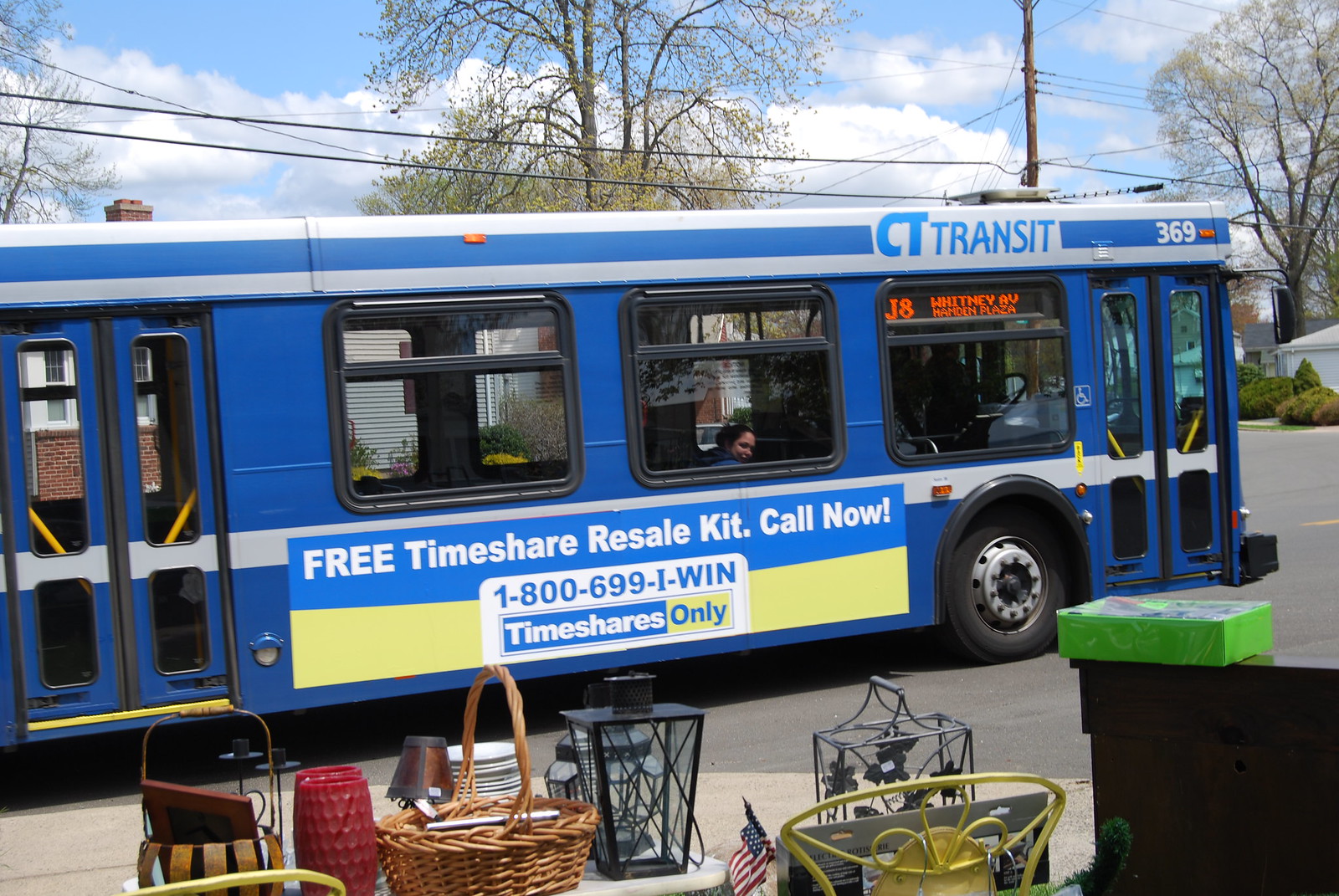In this outdoor daytime photograph, the focal point is a large, medium-blue CT Transit bus prominently positioned in the center of an asphalt road, suggesting a typical urban setting, possibly at a bus stop. The bus features a blue and yellow advertisement on its side and front that reads, "Free Timeshare Resale Kit, Call Now, 1-800-699-I-WIN, Timeshares Only." Above the driver's position, a lit sign indicates the bus route as J8 Whitney Avenue, Handon Plaza. Inside the bus, a female passenger with dark hair and a blue t-shirt is seated near the front, gazing out the window.

In the foreground, there is a circular table adorned with various items, including a brown wicker basket, a black metal and glass lantern, a small American flag, a candle, and some plates. Adjacent to the table are two yellow metal chairs. A black banister with a green square embellishment is also visible nearby. The background of the image features trees, buildings, and telephone poles with power lines stretching across the sky, which is filled with blue hues and fluffy clouds. The scene conjures the essence of a bustling yet serene city street.